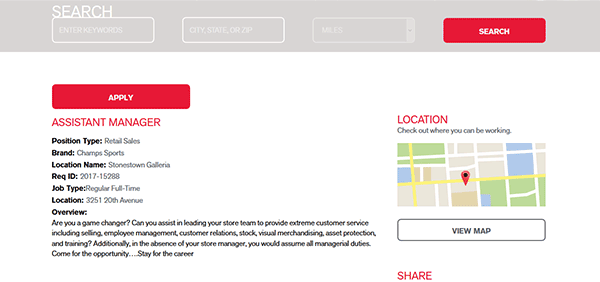This photograph displays a job locator website interface, though the specific website name is not visible as there is no logo present. Dominating the top of the interface is a search bar where users can input keywords related to the job they are seeking. Adjacent to this search bar, there is another input box for entering the city, state, or zip code of the desired job location. A third input box is available, likely for specifying the distance in miles from the entered location, adjacent to which is a prominent red 'Search' button.

Highlighted in the interface is a job listing for an "Assistant Manager" position. The job title "Assistant Manager" is prominently written in red. The position is categorized under "Retail Sales" and is associated with the brand "Champs Sports." The job location is identified as "Stones Town Galleria" with the specific address at "3251 20th Avenue." An ID number for the job is also listed, and the job type is identified as "regular full-time."

On the right side of the interface, there is a box featuring a Google Map, pinpointing the exact location at 3251 20th Avenue. 

The job overview section poses engaging questions to potential applicants, asking, "Are you a game changer?" and outlining responsibilities that include assisting in leading the store team to deliver exceptional customer service, managing employees, handling customer relations, overseeing stock and visual merchandising, asset protection, and staff training. The description notes that in the absence of the Store Manager, the Assistant Manager would assume all managerial duties.

Encouragingly, the final text prompts with a call to action: "Come for the opportunity, stay for the career." Below this overview, there are red buttons to 'Apply' for the job and share the listing, further aiding in the application process.